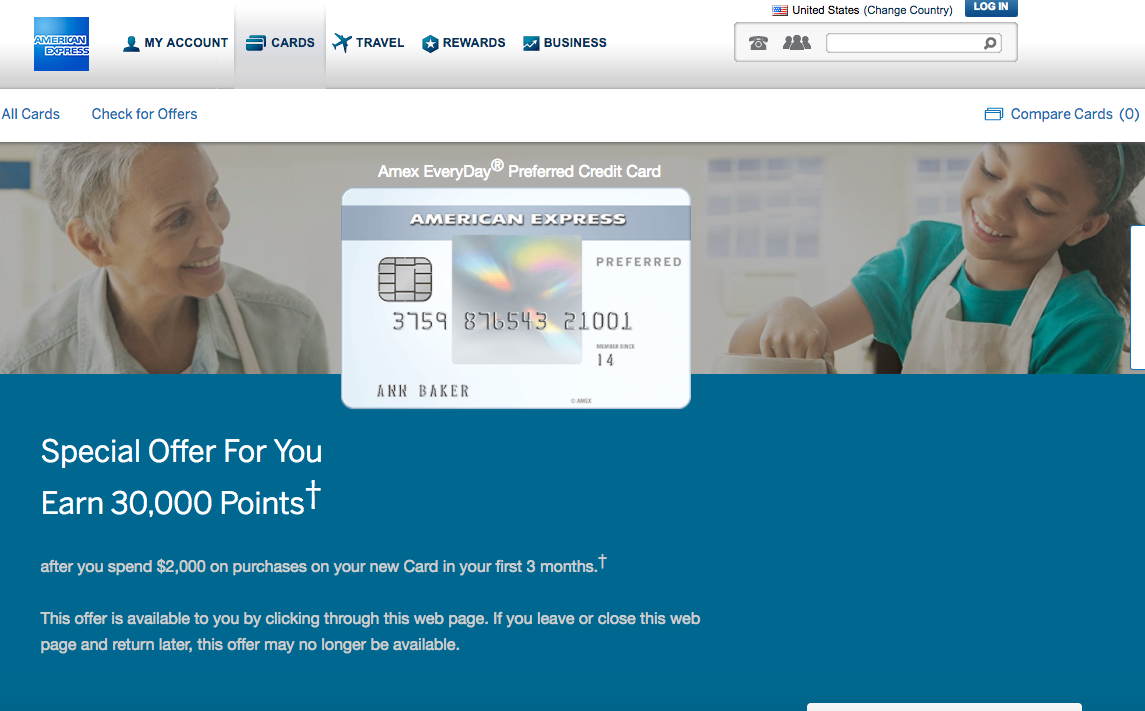The landing page appears to be an American Express promotional webpage, prominently featuring the Amex EveryDay Preferred Credit Card. The card itself is displayed front and center, characterized by a whitish-gray color and issued under the name Ann Baker. The card has an intricate hologram square and the American Express logo imprinted in the middle, adding to its premium look. The card details shown are likely placeholder numbers.

At the top of the page, the American Express logo is visible, accompanied by menu options such as "My Account," "Cards," "Travel Rewards," and "Business." Located in the top-right corner are a search bar in a gray rectangle, an icon depicting a person, and a telephone icon, probably for customer service access. Above these icons, a blue "Log In" button and a United States flag option, which allows users to change their country, are displayed.

Just below the American Express logo, there is a white navigation bar offering options such as "All Cards," "Check for Offers," and "Compare Cards." A note indicates that the current user has zero cards linked to their account.

The background image behind the featured card showcases an older woman with gray hair wearing a light blue button-down shirt and a little girl with dark hair clad in a green shirt, both wearing aprons. They are happily engaged in pottery making, the older woman positioned to the left of the card and the little girl on the right, adding a warm, familial touch to the visual.

Beneath this heartwarming scene lies a blue bar, highlighting a special offer: "Earn 30,000 points." A footnote clarifies that these points are awarded after spending $2,000 on purchases within the first three months of card ownership. It also advises that this offer is accessible only through this specific webpage and may not be available if the webpage is closed or revisited later.

Overall, the webpage aims to attract potential cardholders with visually appealing elements and enticing offers, ensuring clear navigation and essential information readily available.